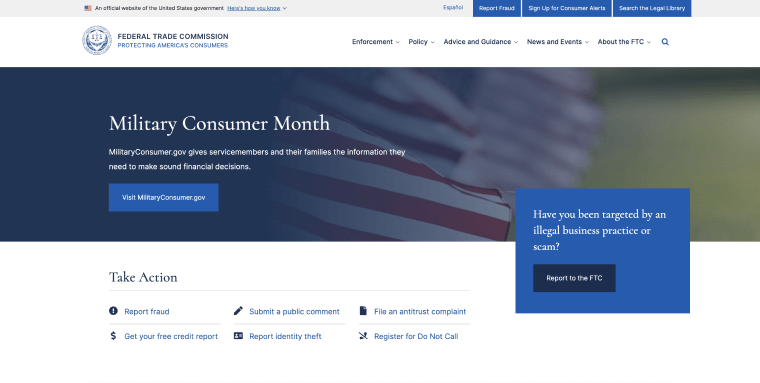This image is a detailed screenshot from the Federal Trade Commission (FTC) website. In the top-left corner, the FTC logo is prominently displayed, featuring the iconic scales of justice encircled by a laurel wreath. To the right of this logo, the text reads "Federal Trade Commission" in bold letters, with the tagline "Protecting America's Consumers" written in smaller, lighter font just below. At the very top of the image is a small American flag with the accompanying text, "An official website of the United States government. Here’s how you know."

The upper right corner features a language option for Español, along with three distinct blue buttons: "Report Fraud," "Sign up for Consumer Alerts," and "Search a Legal Library." Beneath these buttons is a standard navigation menu that includes options for "Enforcement," "Policy," "Advice and Guidance," "News and Events," and "About the FTC," along with a search magnifying glass icon.

The hero image on the main section of the webpage depicts an American flag waving with a graduated blue overlay from left to right, transitioning from solid blue to about 50% transparency, allowing the flag to subtly show through. Large white text on this image declares "Military Consumer Month," with supplementary text stating, "Militaryconsumer.gov gives service members and their families the information they need to make sound financial decisions." A prominent blue button below this text invites users to "Visit MilitaryConsumer.gov."

To the right of the hero image is a semi-transparent box with a blue background. In white text, it asks, "Have you been targeted by an illegal business practice or scam?" Below this, a dark blue button with white text prompts users to "Report to the FTC."

At the bottom-left corner of the image, another section headed by "Take Action," in blue text, lists multiple options: "Report Fraud," "Submit a Public Comment," "File an Antitrust Complaint," "Get your Free Credit Report," "Report Identity Theft," and "Register for Do Not Call." Each option is accompanied by corresponding icons to the left.